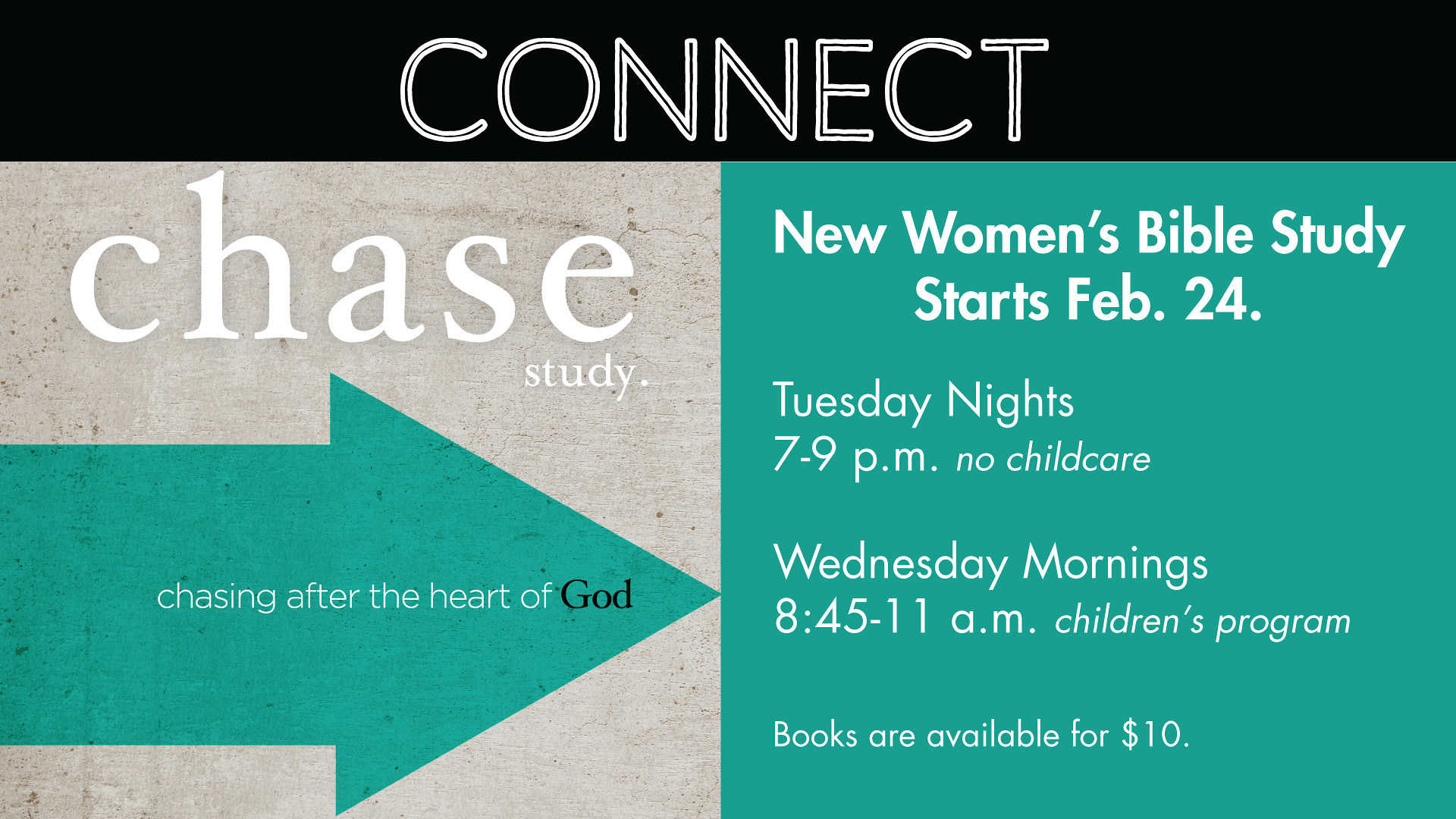The promotional slider image advertises a new women's Bible study event. At the very top, a black banner stretches from left to right, featuring the word "CONNECT" in black text with a white border. The image is divided into two sections. The left section has a gray, cement-like textured background with white text that reads "CHASING STUDY." Over this, a large green arrow points to the right, containing the phrase "chasing after the heart of" in white text, followed by "GOD" in black text. The right section of the image has a solid green background, where white text details the event information: "New Women's Bible Study starts February 24th, Tuesday night 7 to 9 p.m. No childcare. Wednesday mornings 8:45 to 11 a.m. Children's program. Books are available for $10." The image effectively promotes the Bible study event with clear sections, text, and color contrasts.